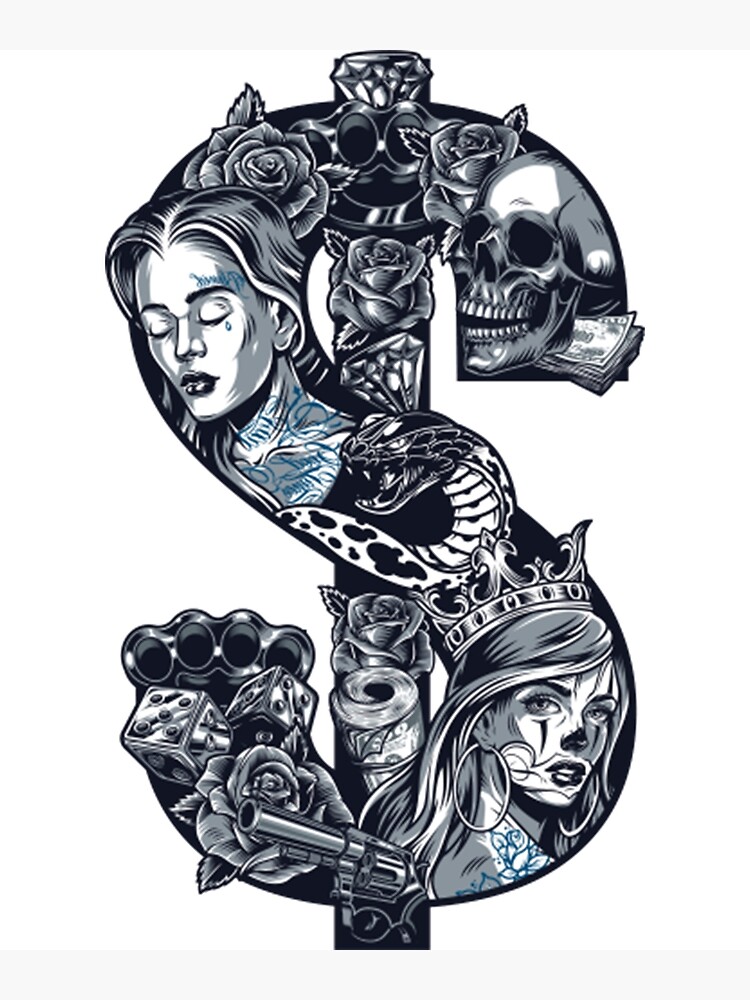The image features a graphic design centered on a large black dollar sign with a single vertical stripe. Most of the design is black and white, with a few blue highlights. Intricately detailed elements adorn the dollar sign, including a human skull with teeth exposed and a slightly open mouth, emitting money from below. Surrounding the skull are multiple black and white roses and a sparkling diamond.

Prominently, a woman’s face appears on the left side of the dollar sign. She has wavy hair down to her ears and her eyes closed, showcasing elaborate tattoos across her neck and chest. A teardrop tattoo in blue rests below her left eye, and additional cursive blue tattooing spans her left eyebrow. Her lips are accentuated with lipstick.

Beneath the woman's face is a threatening black and white cobra with exposed fangs and detailed scales. From here, the image extends to the right with another woman’s face, adorned with a regal crown embedded with gems. She sports long hair past her ears and hoop earrings. Her face is painted with skull-like and clown makeup in black and white tones, and a blue rose tattoo graces her shoulder.

To complete the composition, a black and white revolver, brass knuckles, a pair of dice, and numerous other roses are interspersed around the dollar sign. The lower section of the design features a roll of wadded up dollar bills and another rose, all seamlessly integrated into the graphic, resulting in a visually striking depiction brimming with symbolism and intricate details.